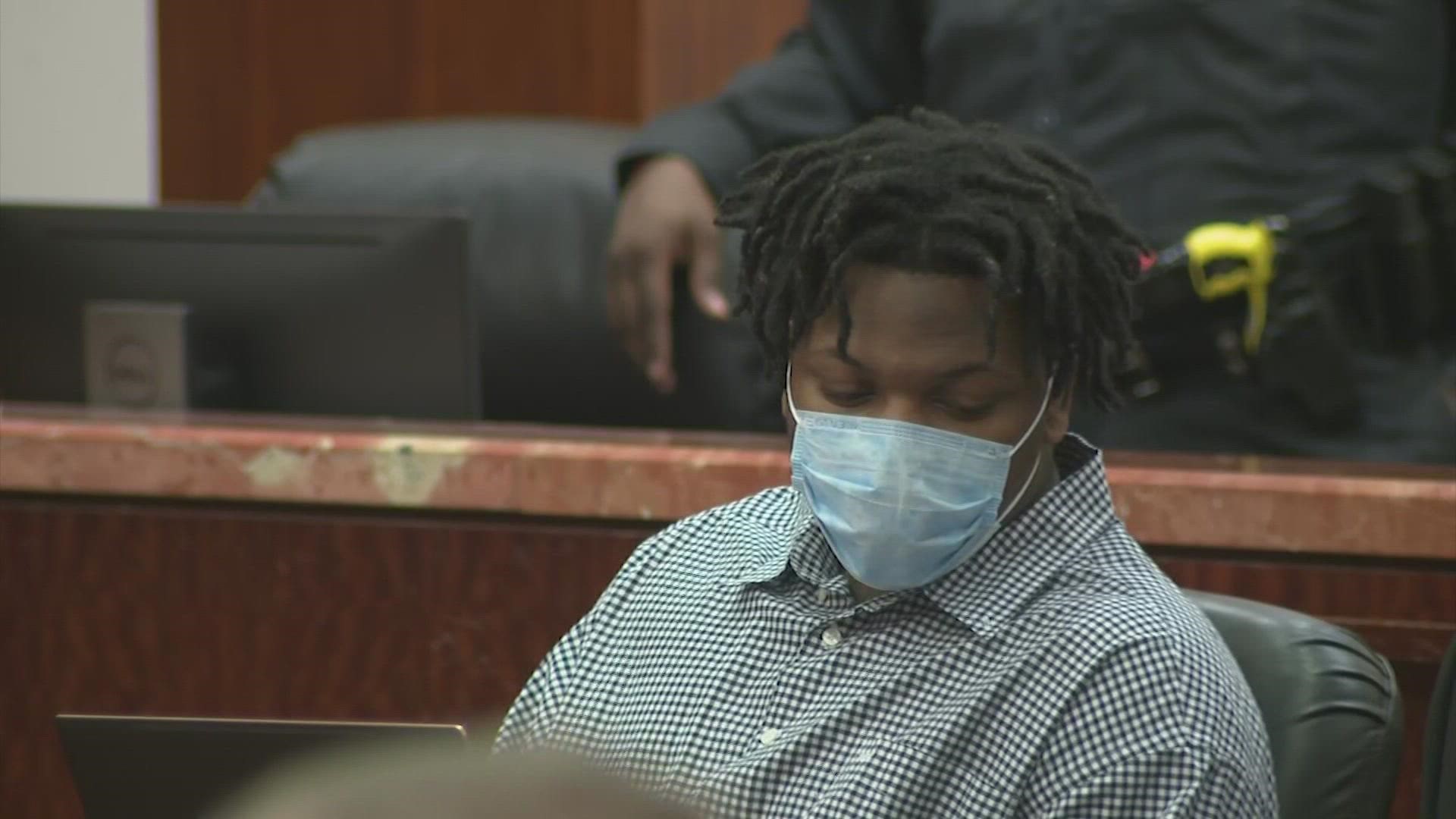This is a detailed photograph capturing a poignant scene inside a courtroom. Central to the image is a young African-American male seated in a black office chair. He is of a stocky build and wears a button-down shirt with a fine gray and white checked pattern. His face is obscured by a light blue surgical mask, and his short dreadlocks cover the tops of his ears. He appears to be looking downward, with his body oriented slightly to the left, giving an impression of deep thought or contemplation.

The courtroom setting around him features a scarred brown wooden bench directly behind him, serving as a backdrop. Further back, to the right, there is a figure of another African-American man in a black uniform, possibly a law enforcement officer, with only his hand, part of his chest, and equipment like a gun belt and a taser visible.

In front of the primary subject, there's a laptop or computer monitor suggesting he may be engaging with a virtual or recorded session. The overall color scheme of the image consists largely of dark grays, blacks, and hints of blue from the face mask, with a subtle pop of yellow from a wristband worn by someone in the background. The scene is lit with indoor lighting, revealing the contrasting elements of the courtroom setting along with the solemn atmosphere, underscored by the COVID-19 pandemic evidenced by the face masks.